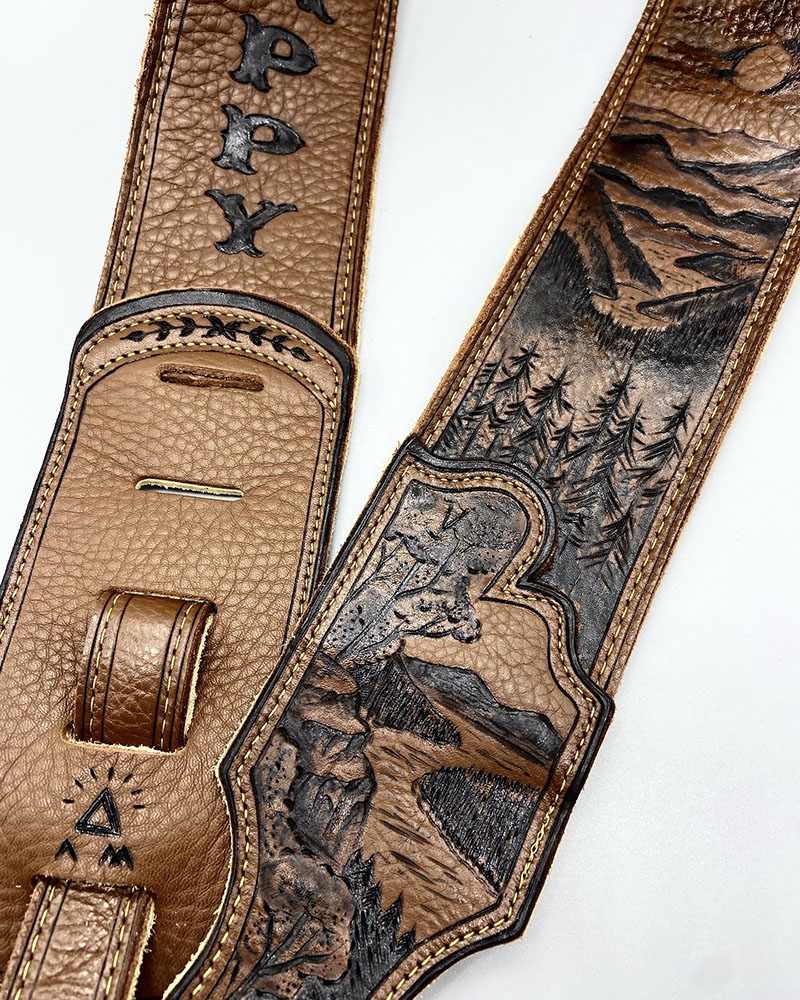This photograph showcases two meticulously crafted leather straps set against a pale background. Both straps appear to be handmade with intricate details highlighting their artisanal quality. 

The left strap, a rich deep brown, bears the engraved letters "P.P.Y." descending the top part of it. Towards its bottom, it features a simple yet elegant design, suggesting a functional aspect with a potential buckle apparatus.

The right strap captivates with its elaborate nature-themed embossing, depicted in a darker, deeper brown shade. It starts with a sun and clouds at the top, followed by a serene mountainous landscape. Below the mountains, a winding river courses through a lush forest of evergreen trees, leading further into an area adorned with more mountains and a dirt path traversing through them. This detailed landscape design captures rivers, valleys, hills, and pine trees, reflecting a harmonious blend of natural elements on a single piece of leather.